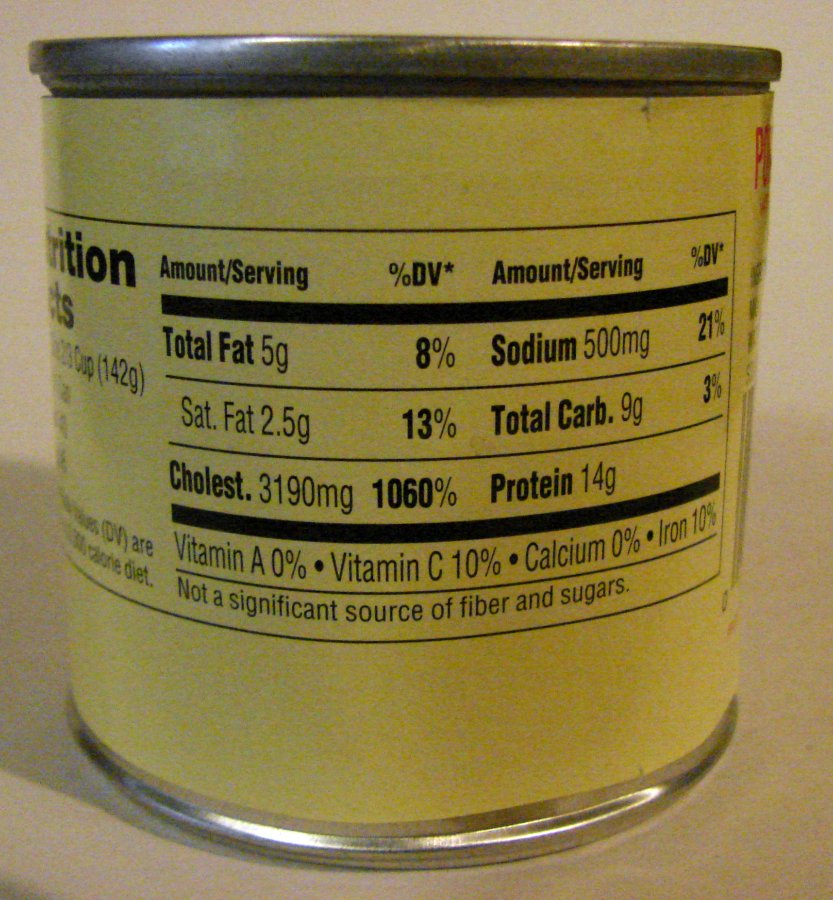A detailed image showcases a solitary canned product, prominently placed against a light peach-colored background. The metallic can, with visible metal rims both at the top and bottom, features a yellow label highlighted with black text. The label is oriented such that the nutrition facts are centered in the frame. Key elements on the label include bold headings like "Amount/Serving" and "Percent DV*", followed by a distinct bold line.

Below this, the label details the nutritional content, listing "Total Fat: 5 grams (8%), Sodium: 500 mg (21%)", along with four additional rows of nutritional information. On the curved right side of the can, there is a glimpse of more text in red, partially visible due to the can's orientation in a landscape fashion. To the left of the can, a shadow is cast, adding depth to the composition. The overall image is notably grainy, enhancing the textured feel of the photo.